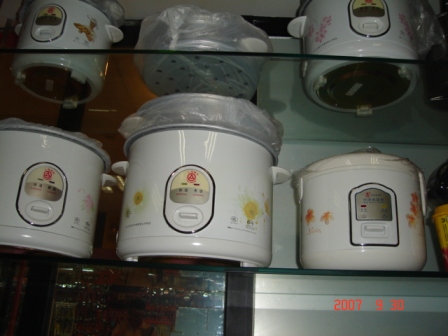The image depicts a display of kitchen appliances, specifically slow cookers, arranged on two glass shelves, possibly in a store. Each shelf holds similarly styled slow cookers, distinguished by their white enamel exteriors and adorned with floral or sunburst designs in shades of gold, yellow, and orange. The bottom shelf features three devices: on the left is a white slow cooker with a central control panel in gold and yellow, a second similar slow cooker with a silver insert wrapped in plastic sitting atop it in the middle, and a smaller version with little orange flowers on the right. The top shelf continues this theme with another white enamel slow cooker on the left, and a silver strainer-like appliance, also wrapped in plastic with holes in the bottom, in the center. To its right is another slow cooker that mimics the ones on the bottom shelf. In the bottom left corner of the image beneath the shelves, there appears to be a dark brown wooden box with some hardware attached, and on the bottom right, a silver box extends behind the appliances. The image appears to have been taken from a low angle, giving a zoomed-in perspective. Additionally, there’s a red timestamp at the bottom of the image indicating "2007 9 30," possibly marking the date September 30, 2007.